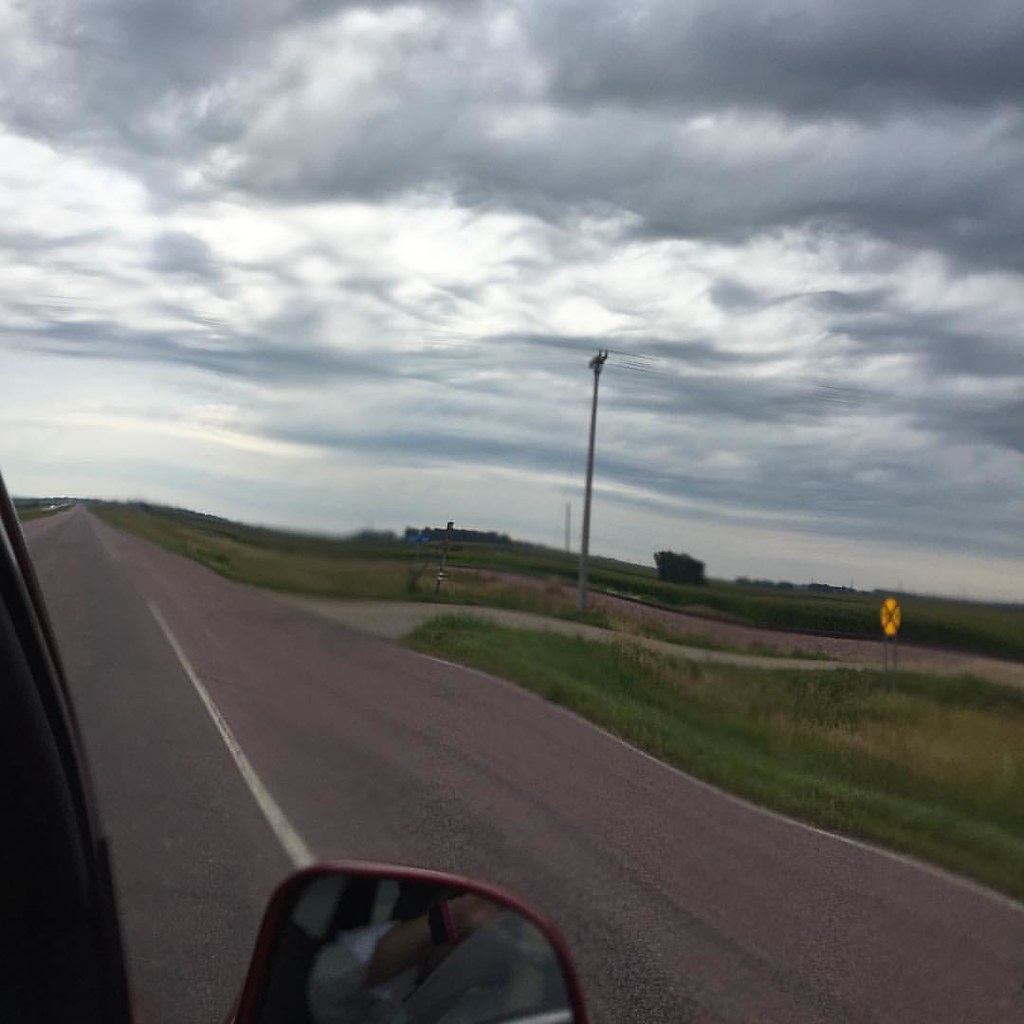This photograph, taken from the passenger side of a moving vehicle, reveals a snapshot of a highway scene viewed from a slightly leaned-out perspective. The right side mirror of the vehicle, rimmed in red, is visible at the bottom of the image, along with a glimpse of the side of the car. The hand of the photographer can be seen in the mirror, adorned with a white shirt and a black and red bracelet. The highway itself is a dark gray, two-lane road with a white line marking the border, and a turnoff area leading to the right. Along the right side of the road, there's a green grassy field with a yellow railroad crossing sign and a tall metal streetlight pole further down. The sky is overcast with thick, ominous gray clouds, casting a gloomy ambiance over the scene. In the distant background, there appears to be a small blue building along with a tree-like object and possibly a large house. The motion blur in the image adds a wavy distortion, emphasizing the movement of the car when the photo was taken.